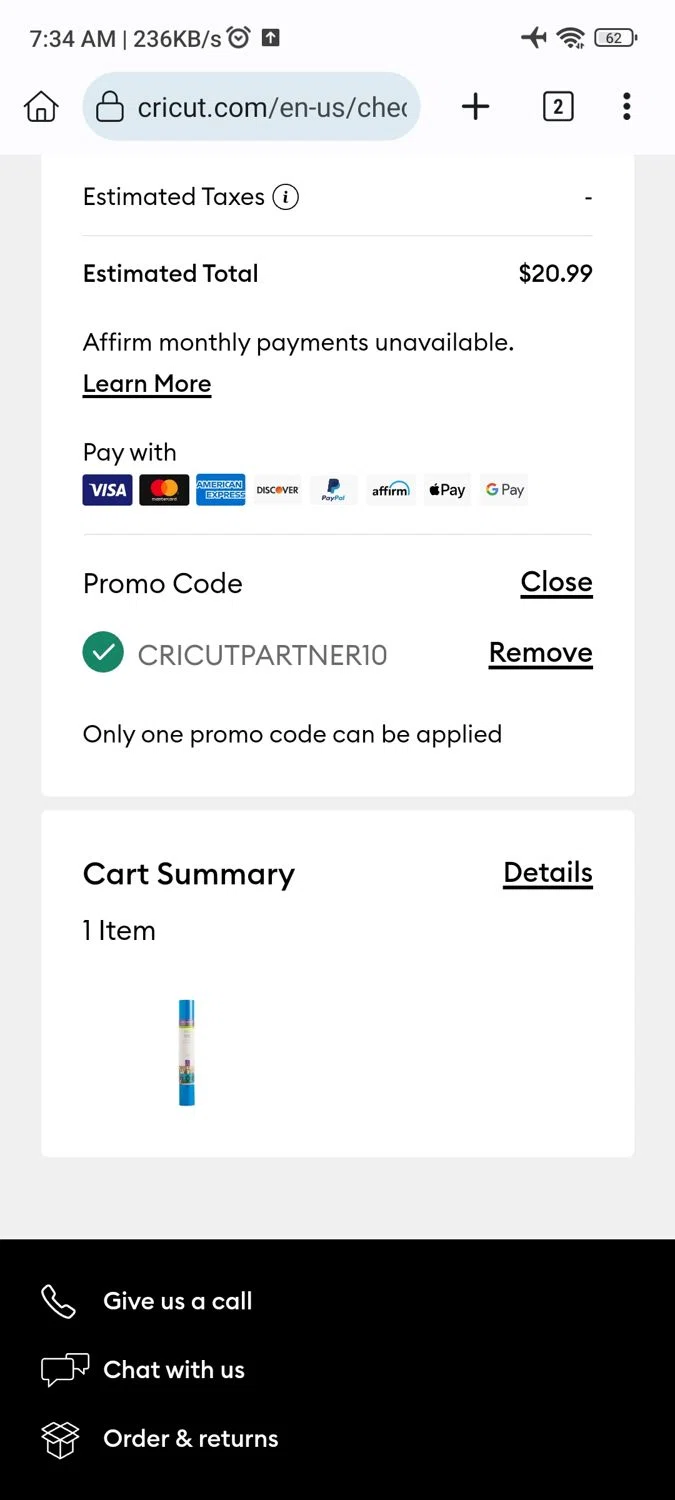Photographic Screenshot of Mobile Device Displaying Cricut.com Checkout Page

In this detailed mobile screenshot taken at 7:34 a.m., a user navigates the Cricut.com checkout page while their phone is in airplane mode. The device shows a connected Wi-Fi signal and a battery life of 62%. At the top of the screen, there’s a home button beside the indication that two web pages are currently open.

The webpage is locked and displays an order summary. The estimated total for the purchase is $20.99, which includes estimated taxes highlighted with an informational button. Below this, there’s an option for monthly payments through Affirm, though it is marked as unavailable at this time. Various payment methods are shown as available, including Visa, MasterCard, Discover, American Express, Affirm, Apple Pay, Google Pay, and PayPal.

A promo code option, "CRICUTPARTNER10," is applied, indicated by a green check mark. There is also an option to remove the promo code, accompanied by a note that only one promo code can be applied at a time.

The cart summary shows one item, with a 'Details' button revealing it to be a blue tube of vinyl.